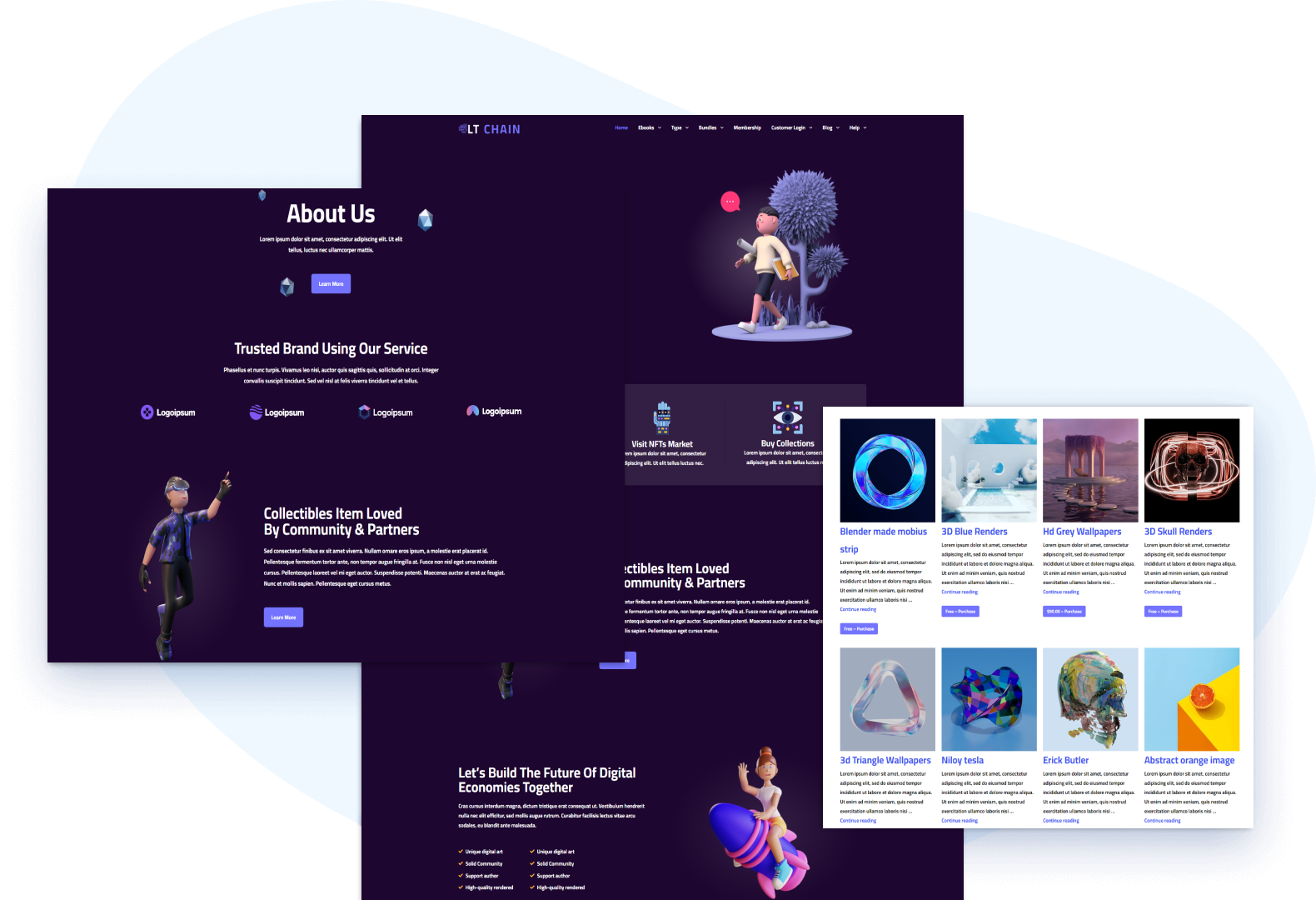This image is a digital collage featuring four distinct sections against a completely black background, highlighting the illuminated content. 

1. The leftmost section is labeled "About Us" and describes collectible items much loved by the community and partners. It emphasizes that they are from a trusted brand and feature a figure resembling a clay model or artwork, pointing upwards with one hand.

2. The next section has the title "LT Chain" at the top, showing a character with a pink speech bubble above them. The character appears animated or crafted from clay, walking by trees. This section reiterates that the collectibles are loved by the community and partners. At the bottom, an animation of a girl riding a rocket is accompanied by the phrase "Let's build the future of digital economies together."

3. The third visible image continues the theme, but detailed visual descriptions are missing as the original information didn't specify this section.

4. The rightmost rectangle is a white area divided into various entries, listing digital assets: Blender-made "Mobius 3D blue renders," HD "Gray wallpapers," "3D skull renders," "3D triangle wallpapers," and names like Nyloi Tesla, Eric Butler, and "Abstract orange images."

Each part of the image composition is meticulously designed to convey a futuristic aesthetic integrated with community-focused branding.